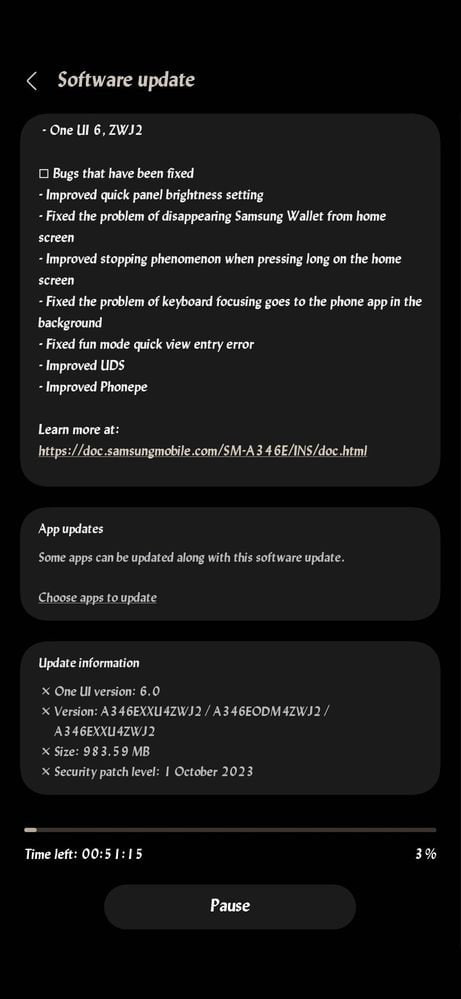This is a screenshot from a cell phone depicting a software update in progress. The background is black with a gray, sideways V-shaped arrow pointing left located about four lines down from the top on the left. To the right of this arrow, bolded white text reads "Software Update." Below this text, three horizontally stacked rectangles with a lighter black background and small white print are included. 

Directly beneath these rectangles, a progress bar is visible. On the left side of this bar, there is a white minus sign. The bar itself is light gray, indicating the progress of the update. Below the progress bar, white text displays "Time Left 00:51:15," indicating the remaining time for the update. To the right of this line, the screen shows "3%" to indicate the current progress percentage.

A couple of lines below this information, an oval-shaped button with a light black or dark gray background is centered. In the middle of this button, bolded white text reads "Pause," giving the user the option to pause the update.